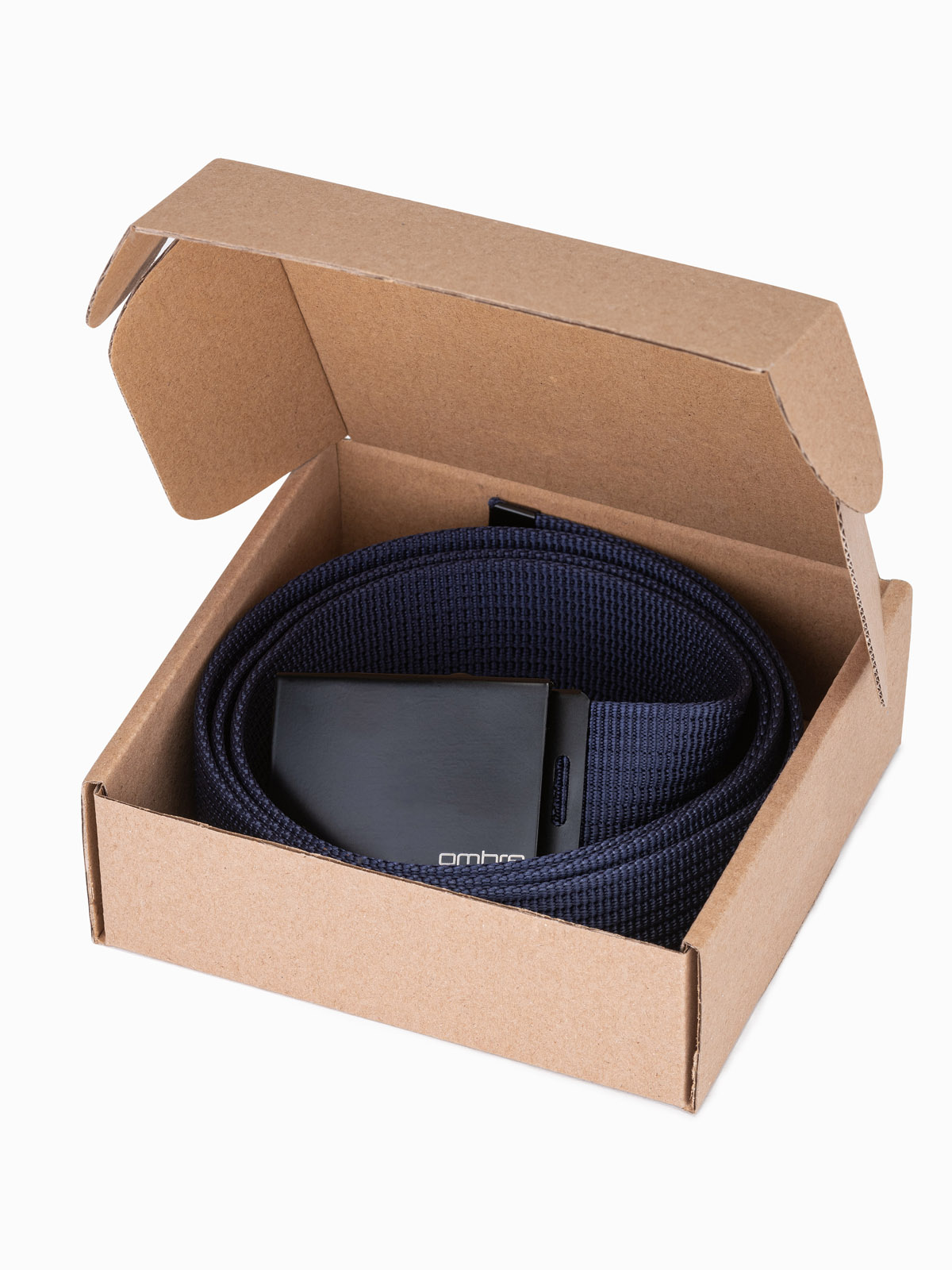This photograph showcases a men's fabric belt neatly coiled inside a small, plain cardboard box. The belt, likely made of canvas and finely interwoven, comes in a dark hue, possibly navy blue or dark gray, and features a smooth, black metallic buckle. This buckle appears to be one-size-fits-all and carries a partially visible logo, "OMBRE," in small white lettering. At the belt's end is a metal tag to prevent fraying. The cardboard box, approximately 6 inches square and 3 inches tall, is brown and nondescript, with tabs that lock to close it. The image, likely from an advertisement, is set against a minimalistic off-white background, ensuring the product stands out.